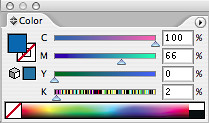This image is a small, rectangular thumbnail screenshot of a photo editing program, specifically on an Apple Mac computer. The graphic showcases a user interface element of the software, representing a color management sub-menu for controlling CMYK values in a color palette. At the top of the screenshot, there's a tab labeled "Color." Directly below this is a blue square displaying the current selected color. Adjacent to this, on the left, are gradient sliders labeled with CMYK (Cyan, Magenta, Yellow, Black) for adjusting the respective color percentages. Each slider is accompanied by numeric values, showing precise color adjustments. At the bottom of the interface, there is a thicker, elongated rainbow dial, allowing users to select the desired color range. The interface presents a way to fine-tune colors, likely used for tasks in photo editing or painting software.